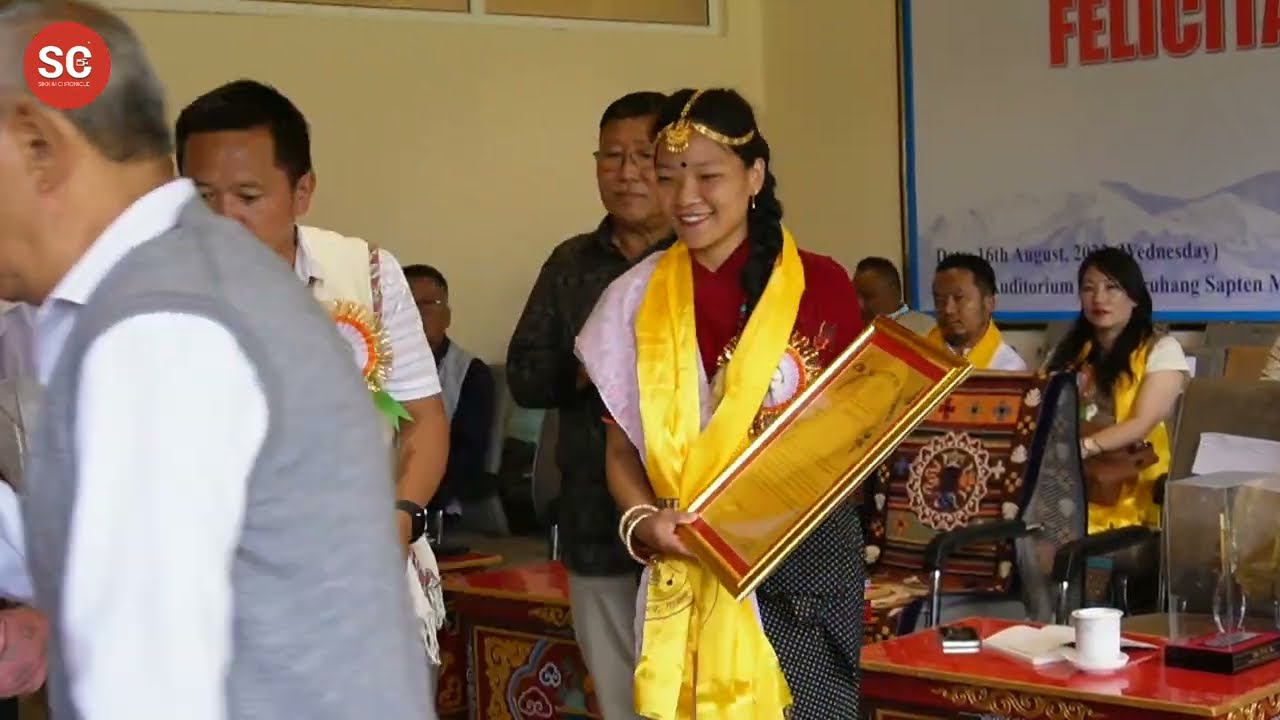The image depicts an indoor event, likely an award ceremony or graduation, characterized by a vibrant and bustling atmosphere. Central to the composition is a smiling woman dressed in an eye-catching red, white, and yellow outfit adorned with a bright golden-yellow scarf and a decorative golden hairpiece. She proudly holds a large framed picture, possibly an award or certificate.

Surrounding her are several other individuals: to her left stands a man in a gray vest with white long sleeves, and behind him is another man wearing a white short-sleeve shirt decorated with a sun and flower pattern, his shirt trimmed in gold. On her right, we see another woman with a bright yellow scarf, and next to her is a man dressed in a black shirt and white pants. In the background, three seated individuals also wear yellow scarves, adding to the ceremonious feel.

The room itself is detailed with décor and various items: multiple tables draped in red and decorated yellow accents, all holding items like cups, a mobile phone, an open book, and a vase (possibly also an award). One wall in the background is beige and adorned with a large poster, which features partial readable text "FELICI...," a picture of a mountain range, and remnants of a date with “16th August” and “Wednesday, auditorium” visible. A logo in the upper left corner of the poster reads "SC" in white lettering within a red circle. The event space is well-lit, allowing the detailed and colorful decorations and attire to stand out vividly.